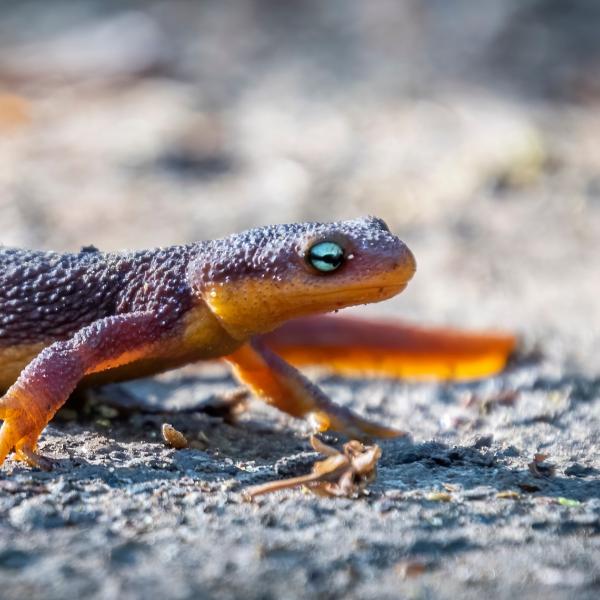The image is a very close-up photograph of a small lizard, centrally positioned on a sandy gray, slightly pebbled ground. The lizard's vibrant coloration features a striking mix of hues: the head and upper body possess shades of purple, the legs exhibit light purple and yellow tones, and the underside glows with yellow-orange hues. Its back appears rough and transitions to a dark gray or black tint. Intriguingly, its long tail, which stretches behind the lizard, displays an intermingling of red and yellow shades, though it is out of focus. In sharp contrast, the lizard's eyes stand out with their light blue irises and black pupils, capturing attention against its vividly colored body. The photograph highlights these eyes, head, arms, and back in clear focus, while the tail and background remain softly blurred, emphasizing the creature's intricate details.